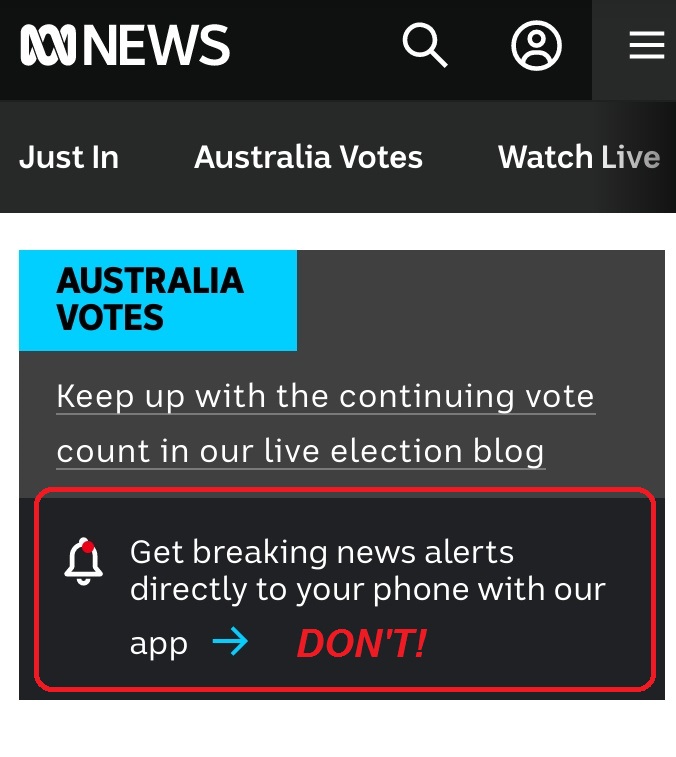The image is a small, simplistic graphic primarily in black, gray, and white hues. At the top, a solid black border spans three-quarters of the width, transitioning into a gray block containing three horizontal white lines, presumably an options button. Within the black section, there are three icons: a profile image icon, a white magnifying glass symbolizing search, and a logo displaying an 'N' that loops back on itself resembling an infinity symbol, labeled 'News'.

Beneath this, a gray banner highlights “Australia votes” alongside the prompt to “watch live.” In the primary section of the image, a blue box in the upper left corner reiterates “Australia votes.” Adjacent to this, on a gray background with white text, it states, “Keep up with the continuing vote count in our live election blog.”

Toward the bottom, a red, digitally added box frames a notification bell icon in white with a red dot, accompanied by the message: “Get breaking news alerts directly to your phone with our app. Don't.”